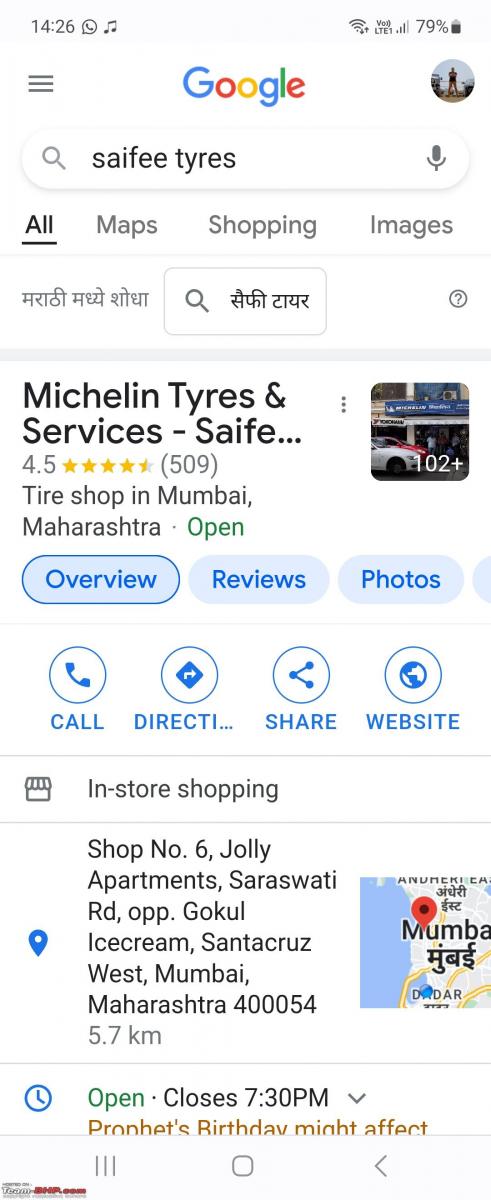**Detailed Screenshot Description:**

This image is a screenshot of a Google search performed on a mobile device, captured at 14:26 with the device battery at 79%. The search query entered is "Saifee Tyres," spelled specifically as "S-A-I-F-E-E T-Y-R-E-S."

The search results prominently display a business named "Michelin Tires and Services" located in Mumbai, India. This establishment boasts an impressive 4.5-star rating based on 509 reviews. Below the business name, there are navigation tabs including "Overview," "Reviews," and "Photos."

Further down, additional action buttons are available which allow the user to "Call," get "Directions," share the establishment, or visit its website. The business offers in-store shopping services.

The address provided for Michelin Tires and Services is:
Shop Number 6, Jolly Apartments,
Saraswati Road, near Gokul Ice Cream,
Santa Cruz West,
Mumbai, Maharashtra, 40054.

The shop is 5.7 kilometers away from the user's current location and is currently open, with operating hours until 7:30 PM.